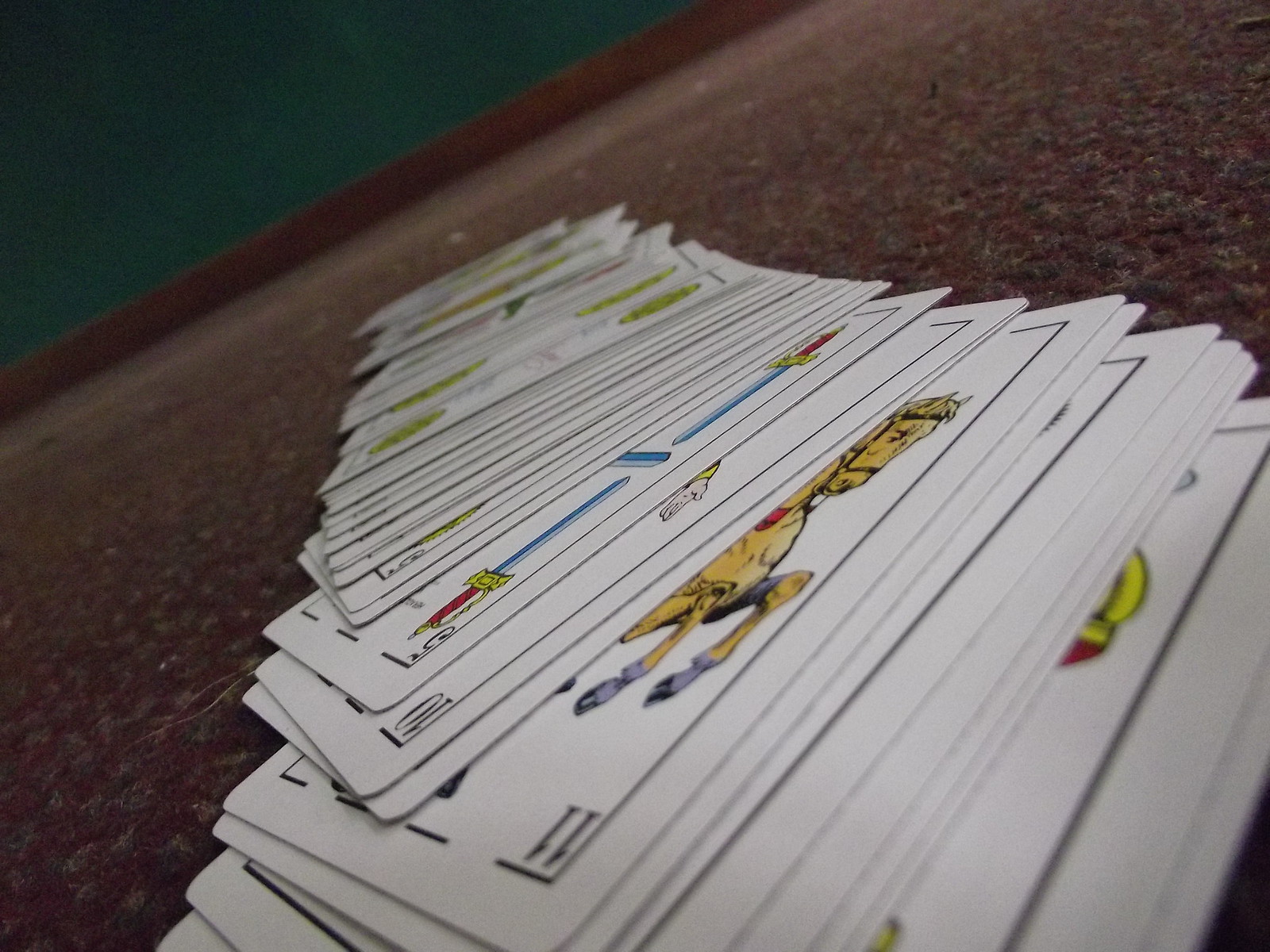A striking deck of cards is prominently displayed in this image, offering a glimpse into its unique design. The background of the image is divided diagonally; the top left corner is shrouded in black, forming a slanting line that runs from the center-left up to off-center right, juxtaposing against a darker brown background that is subtly speckled with lighter brown spots.

The deck is artistically fanned out on the bottom right and spread upwards towards the top left corner, showcasing its distinctive appeal. Unlike typical modern playing cards, these cards feature a set of graphics that are both artistic and ornate, reminiscent of tarot card illustrations rather than the conventional faces found on a standard Bicycle deck.

Each card face is white with a thin black border outlining the decorative elements. The numbers in the corners are written in a fine, black typeface and lack any traditional suit symbols such as clubs, spades, hearts, or diamonds, further emphasizing their unique aesthetic.